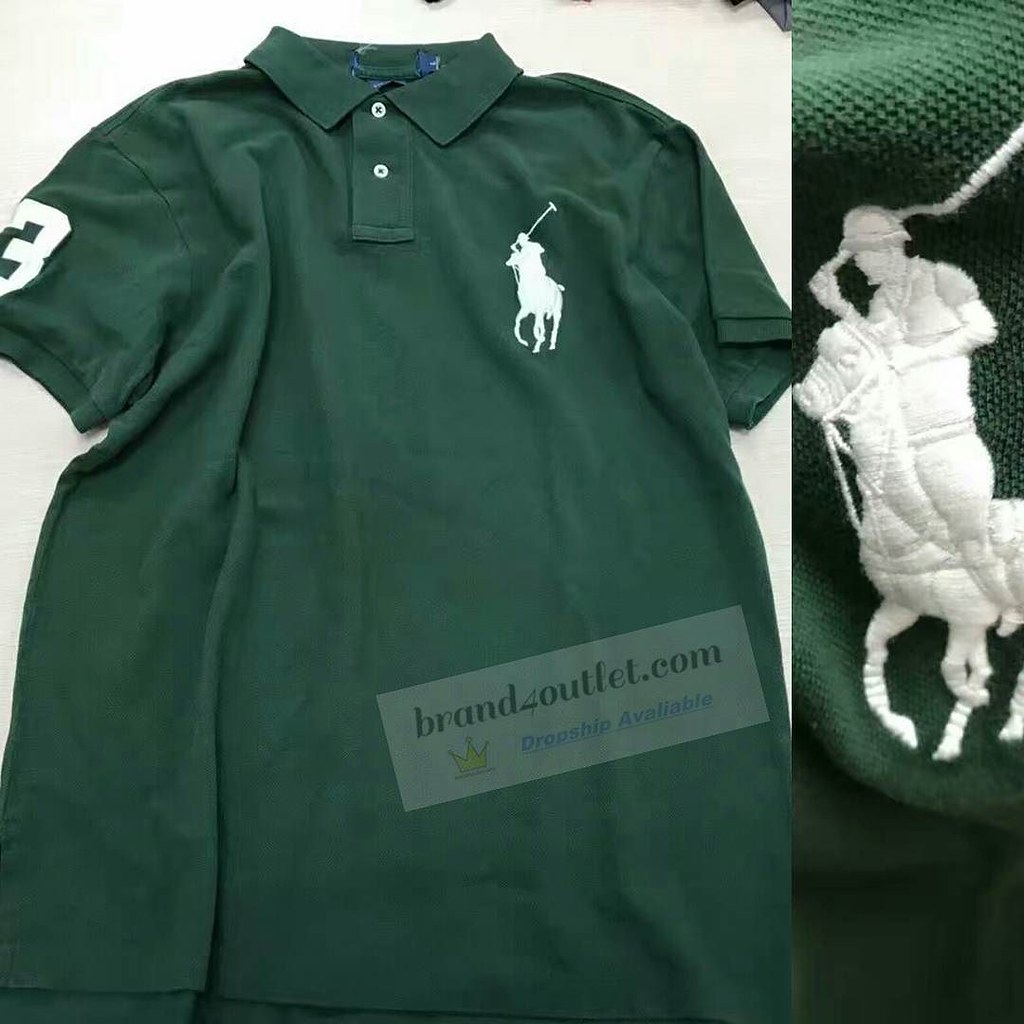This is a detailed photograph of a dark forest green polo shirt, prominently displayed against a white background. The shirt features a neatly folded collar and two white plastic buttons with green thread near the neck, which are characteristic of a classic polo design. The short-sleeved garment has a large embroidered number "3" on the right arm sleeve, adding a distinct sporty touch. On the left chest, there is an intricately embroidered logo depicting a stylized image of a polo player on horseback, poised with a polo stick raised. This meticulous stitching enhances the official look and feel of the shirt. The texture of the fabric is visible, showcasing the traditional, durable weave associated with polo shirts. Overlaid on this image is a semi-transparent white rectangle bearing the text "brandforoutlet.com" in black, accompanied by the statement "Drop Ship Available" in blue, framing the image as an advertisement for this website that offers authentic polo apparel.